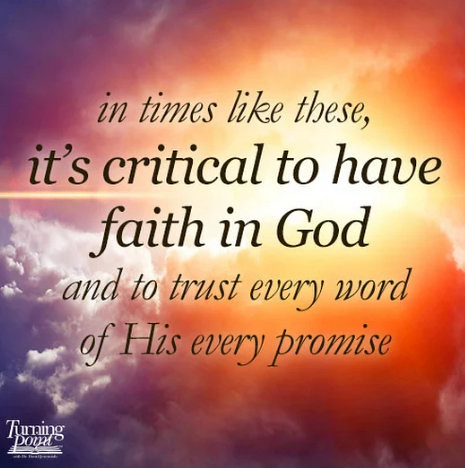The image presents a breathtaking sky painted with a mesmerizing palette of light orange, dark orange, yellow, purple, and white, creating a heavenly scene. Puffy white clouds float near the bottom left, while the upper left corner boasts dark blue clouds. At the center of the image, written in an elegant cursive font, black text conveys an inspiring message: "In times like these, it's critical to have faith in God and to trust every word of His every promise." The quote stretches over five lines, with the second line, "it's critical to have faith in God," emphasized in bold and a slightly larger typeface. The first, third, and fourth lines differ in type set from the bolded second line. At the bottom left corner, a small logo resembling an open book with the words "Turning Points" is subtly placed. This caption integrates the visual harmony of the scene with the uplifting text, highlighting the importance of faith and trust.